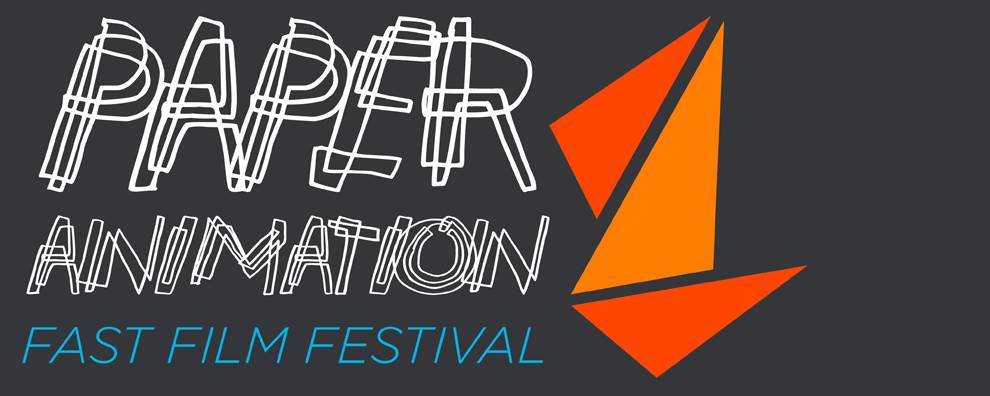This image displays a film festival flyer set against a long, black rectangular background. Dominantly on the left side, it features the title "Paper Animation" in a distinct 3D pencil font styled with white text. This title appears as if it's scribbled multiple times, creating a static-like visual effect. Beneath it, "Fast Film Festival" is written in a clean, blue font. To the right of this text lies a logo composed of three triangles, arranged to form a stack. These triangles vary in shades of orange, with two darker orange ones and one light orange, positioned in multiple directions both vertically and horizontally. The overall layout keeps the right side relatively empty, drawing attention to the striking elements on the left and the logo in the middle.